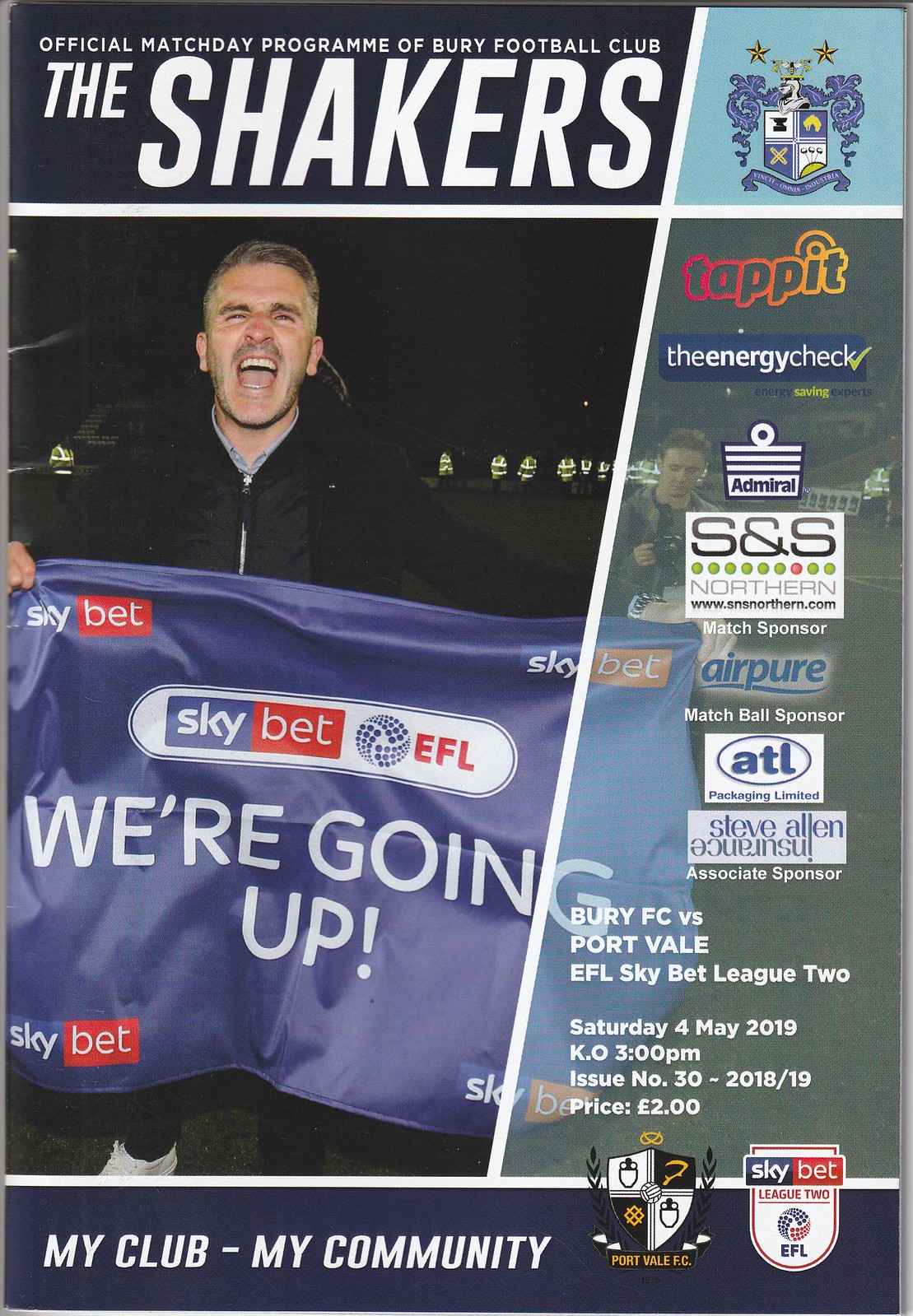The image depicts the official match day program for Bury Football Club, known as "The Shakers," for a soccer game against Port Vale. At the top, in bold white letters on a black background, it reads "Official Match Day Program of Bury Football Club, The Shakers." On the upper right corner, there's the team's emblem set against a light blue backdrop. The main part of the image features a man with his mouth open, as if yelling, holding up a blue flag that says "Sky BET," "We're Going Up." Beside him, partially obscured by printing, stands another man. Down the right side of the program cover, various sponsor names are listed, such as Tap It, Energy Check, Admiral, SNS Northern, Air Pure, ATL, and Steve Allen. Beneath the man's image, it states the details of the match: "Bury FC vs. Port Vale, EFL Sky BET League 2, Saturday 4 May 2019, KO 3 p.m., Issue Number 30, 2018-19, Price £2.00." At the bottom, in white letters on a blue strip, it says "My Club, My Community." Also at the bottom are two badges: the Sky BET League 2 EFL logo on the right, and the Port Vale FC badge.